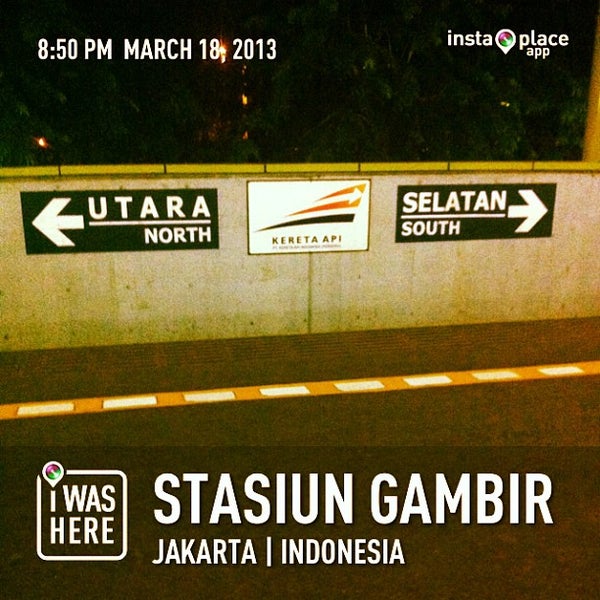The image is a screenshot from a game, displaying a scene resembling a road or railway alongside a cement wall. At the top left corner, the timestamp "8.50pm March 18th, 2013" is shown in white, capitalized text. The top right corner features the InstaPlace app logo. The background of the image includes digitally created treetops and scattered lights. On the cement wall in the middle of the image, two directional signs are visible: "Utara North" with an arrow pointing left and "Salatin South" with an arrow pointing right. In the center, a sign reads "Kereta API" with a flag symbol above it. The foreground shows the road or railway marked with an orange and white striped line, and a yellow section atop the wall. At the bottom of the image, the text "I was here," with a distinct logo dotting the 'I', appears followed by "Stasiun Gambir Jakarta Indonesia," all in white text.